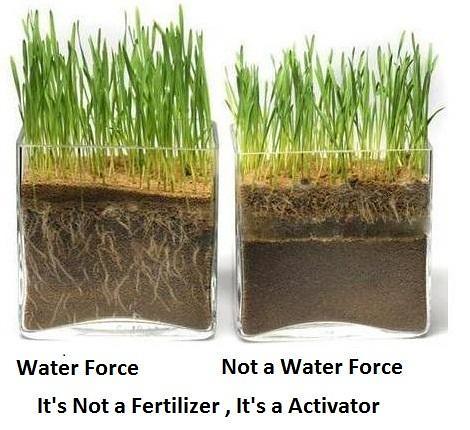The image displays two side-by-side rectangular glass containers filled with brown soil and grass, clearly visible through the transparent glass. The container on the left features robust roots extending all the way to the bottom, with taller green grass emerging from the top; this container is labeled "water force." The container on the right, labeled "not a water force," contains shorter grass with no visible roots. Both containers bear an additional label stating, "it's not a fertilizer, it's an activator." The overall background is stark white, emphasizing the glass containers with their distinct differences in grass growth and root development.